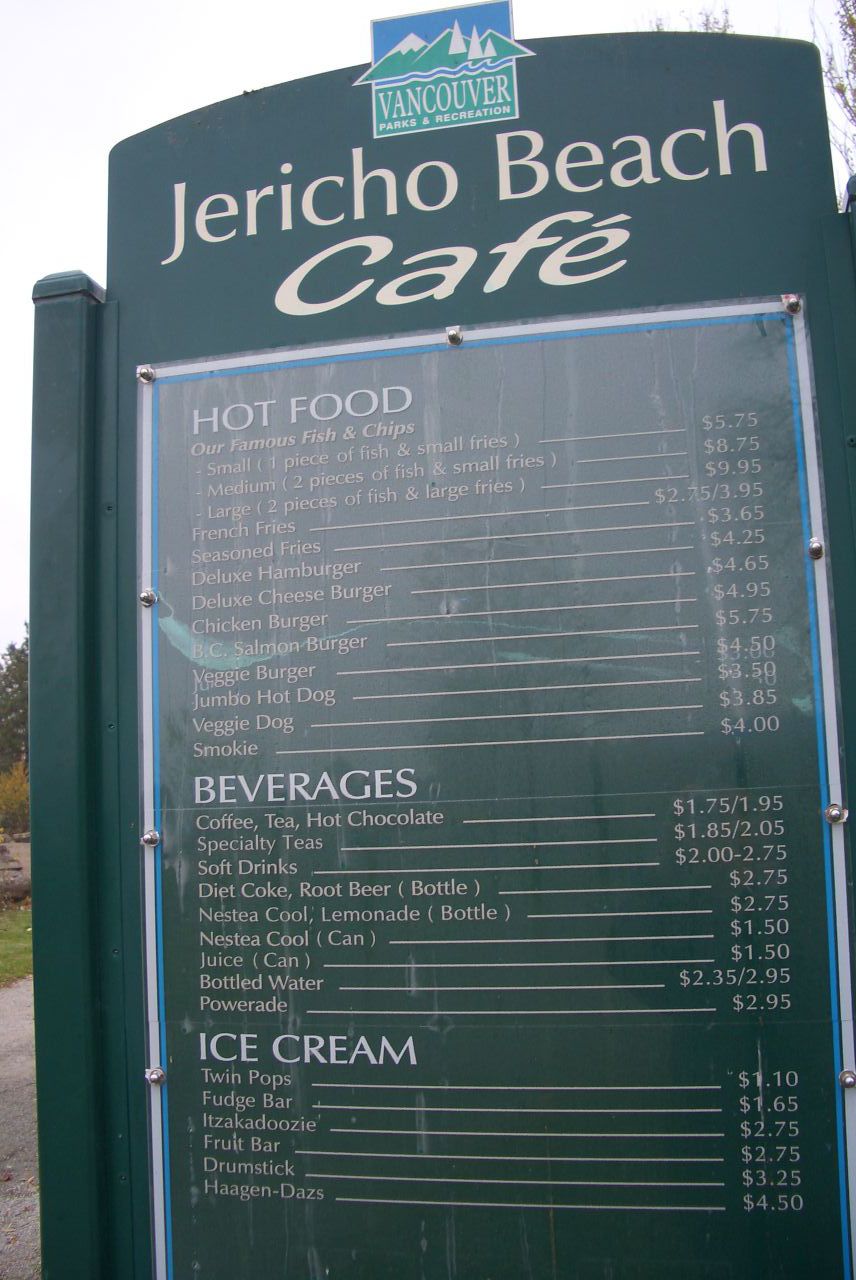In this vertically oriented image captured under natural daylight, the scene unfolds with a light, mostly colorless sky forming the horizontal upper background. On the left edge, a small segment shows a strip of concrete at the bottom, ascending into a patch of grass and a solitary tree. Dominating the frame is a prominently situated restaurant sign, vertically rectangular with an elegantly curved top. The sign is a deep, dark green adorned with pristine white lettering that reads "Jericho Beach Cafe" at the top. Below this, a sizable section of clear plexiglass reveals the cafe's menu, albeit partially obscured by glare. The menu is meticulously detailed, beginning with a "Hot Food" category listing approximately a dozen items, each accompanied by corresponding prices on the right. Following are the "Beverages," similarly itemized with prices. Concluding the menu, the "Ice Cream" category features several selections, each also paired with their respective prices.